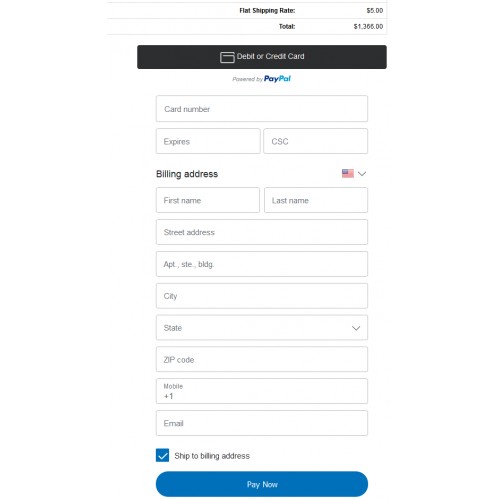The detailed caption for the image under the "Websites" category can be formulated as follows:

"This image depicts a minimalistic payment page layout. At the very top of the page, there is a message stating 'Flat Shipping Rate $5.00', followed by another line that reads 'Total $13.66'. Below these, a black line displays the option 'Debit or Credit Card'. Underneath this line, the text 'Powered by PayPal' is visible. The form includes several blank boxes for inputting payment details: 'Credit Card Number', 'Expires', and 'CVC'. 

Further down the page, the form requests the 'Billing Address', accompanied by an American flag icon with a drop-down menu beside it for selecting the country. The form then provides a series of blank boxes for 'First Name', 'Last Name', 'Street Address', 'Apartment/Suite/Building', 'City', 'State', 'ZIP Code', 'Mobile Number', and 'Email'. 

At the bottom of the form, a checkbox labeled 'Ship to billing address' is ticked and highlighted in blue, indicating this option is selected by default. Finally, an oval button at the bottom center of the page reads 'Pay Now', allowing users to complete their purchase."